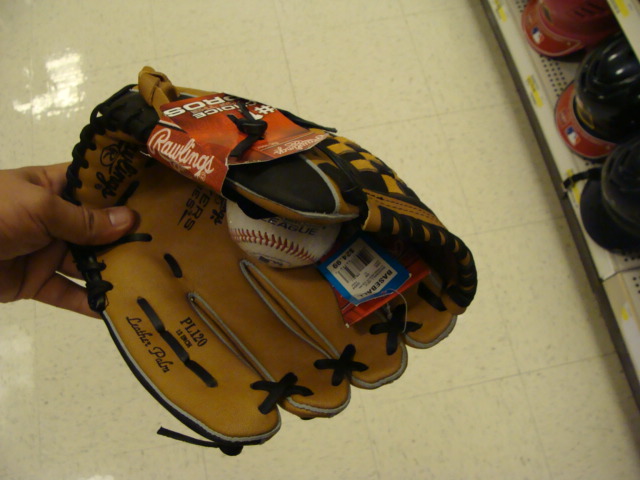This color photograph features a new Rawlings baseball glove prominently in the center, occupying about 60 to 70% of the image. The glove is held by a hand with medium dark skin entering from the left. The glove itself has a yellow interior and multicolored exterior, including light brown, dark brown stitching, and grey cords forming Xs between the fingers. It displays multiple tags, including a blue label with a white square, a red tag with white writing, and possibly some text that resembles "Pluto" and "R-O-S" upside down. The glove also holds a baseball with red stitching inside.

The background of the image appears to be a cream-colored tiled floor with black lines, possibly within a store. In the upper right-hand side of the image, there is light reflecting off the tiles, and a metallic display shelf extends from the top to the bottom right corner. This shelf holds a row of baseball hats or hitter's helmets, with the top object being red, the middle one black with a red brim, and the bottom one black, all showing official NBA stickers, indicating they may be used.